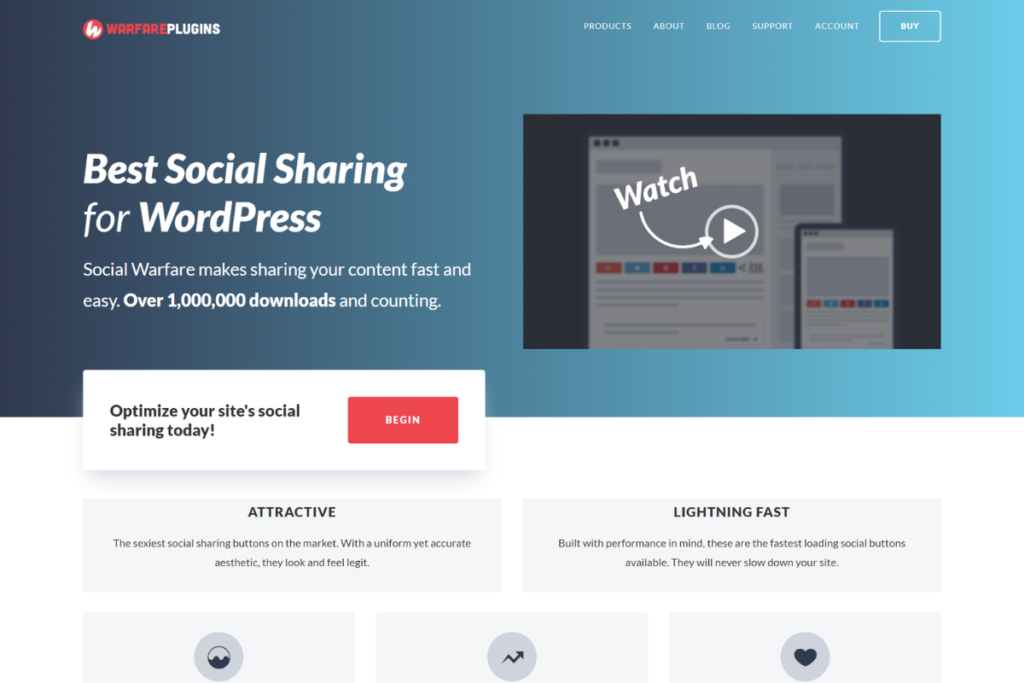The image is a left-to-right horizontal graphic that appears to be sourced from a website, accessible via computer or smart device. The background is a gradient of blue-green, starting darker on the left and transitioning to a lighter shade on the right, adding depth without any distinct texture. In the upper left corner, there's a small red circle with a white "W" inside. Next to it, the text "Warfare" in red and "Plugins" in white appears.

On the top right, there's a navigation menu featuring the options: Products, About, Blog, Support, Account, and a prominent "Buy" button enclosed in a rectangle.

Below this header, on the left side, the text reads, "Best social sharing for WordPress" in a large font. Smaller text underneath states, "Social Warfare makes sharing your content fast and easy—over 1 million downloads and counting."

To the right of this text, there is an embedded video thumbnail featuring a screenshot of web pages. A play button with an arrow invites users to watch the video. The video's caption reads, "Optimize your site's social sharing today." Beneath this, a red button labeled "Begin" is available for users to start optimizing their social sharing.

At the bottom of the image, additional information highlights the attractiveness and speed of the service, followed by a series of circular buttons with black icons, presumably for additional functionalities or social media integrations.